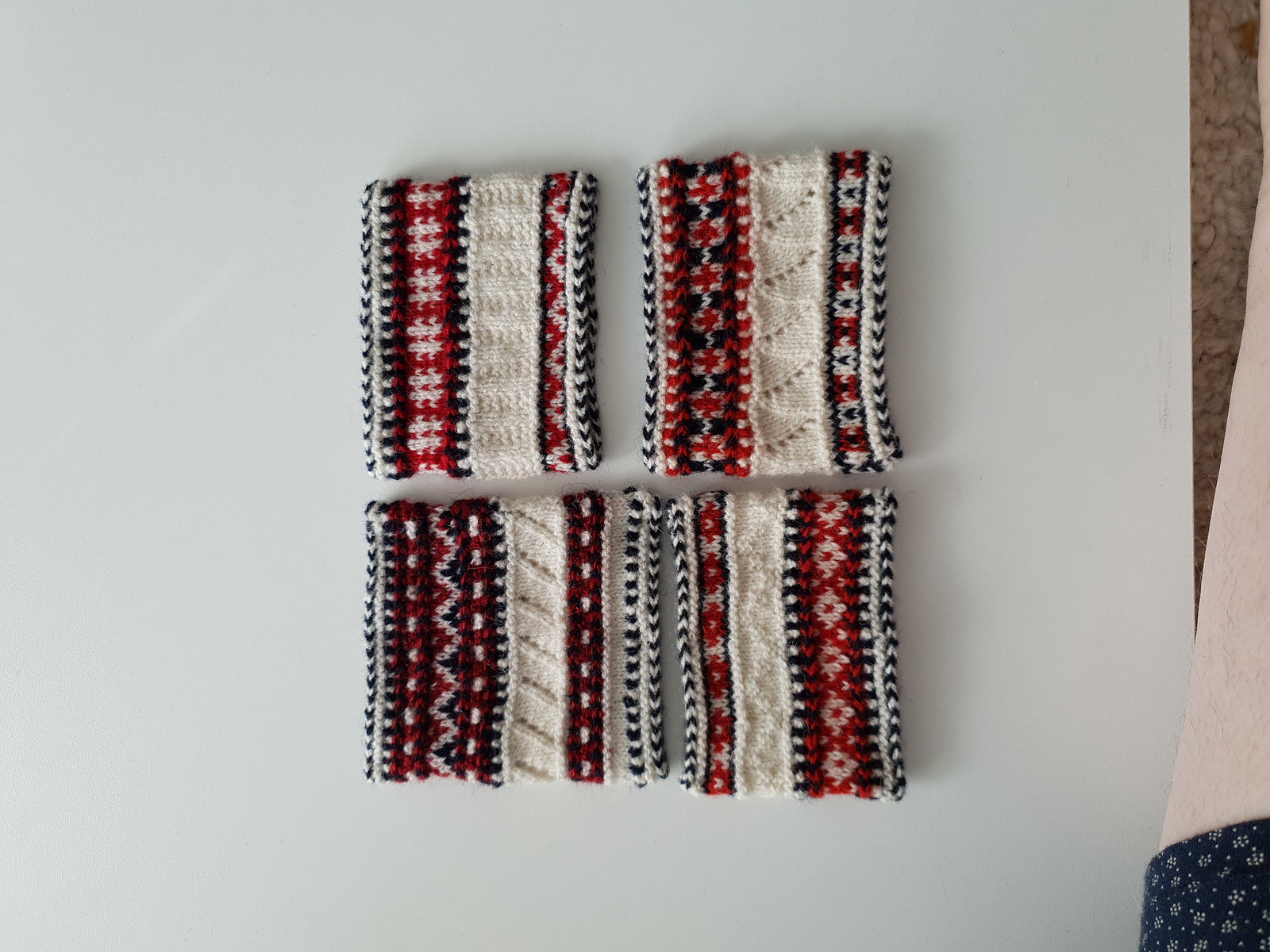This is a close-up photo set on a white table surface, partially visible against a brown-beige carpet backdrop. The image showcases four hand-knitted winter accessories, likely head or wrist warmers, crafted in intricate red, white, and black patterns. These knitted pieces, featuring varying designs such as stripes, checkered, and bars, are neatly laid out in a 2x2 arrangement. Each piece, while maintaining a common color scheme and theme, offers unique details, indicative of meticulous work. The photo is in focus but somewhat dimly lit. Additionally, on the right edge of the image, a pale human leg is visible, dressed in blue shorts adorned with white flowers, hinting at a relaxed indoor setting.